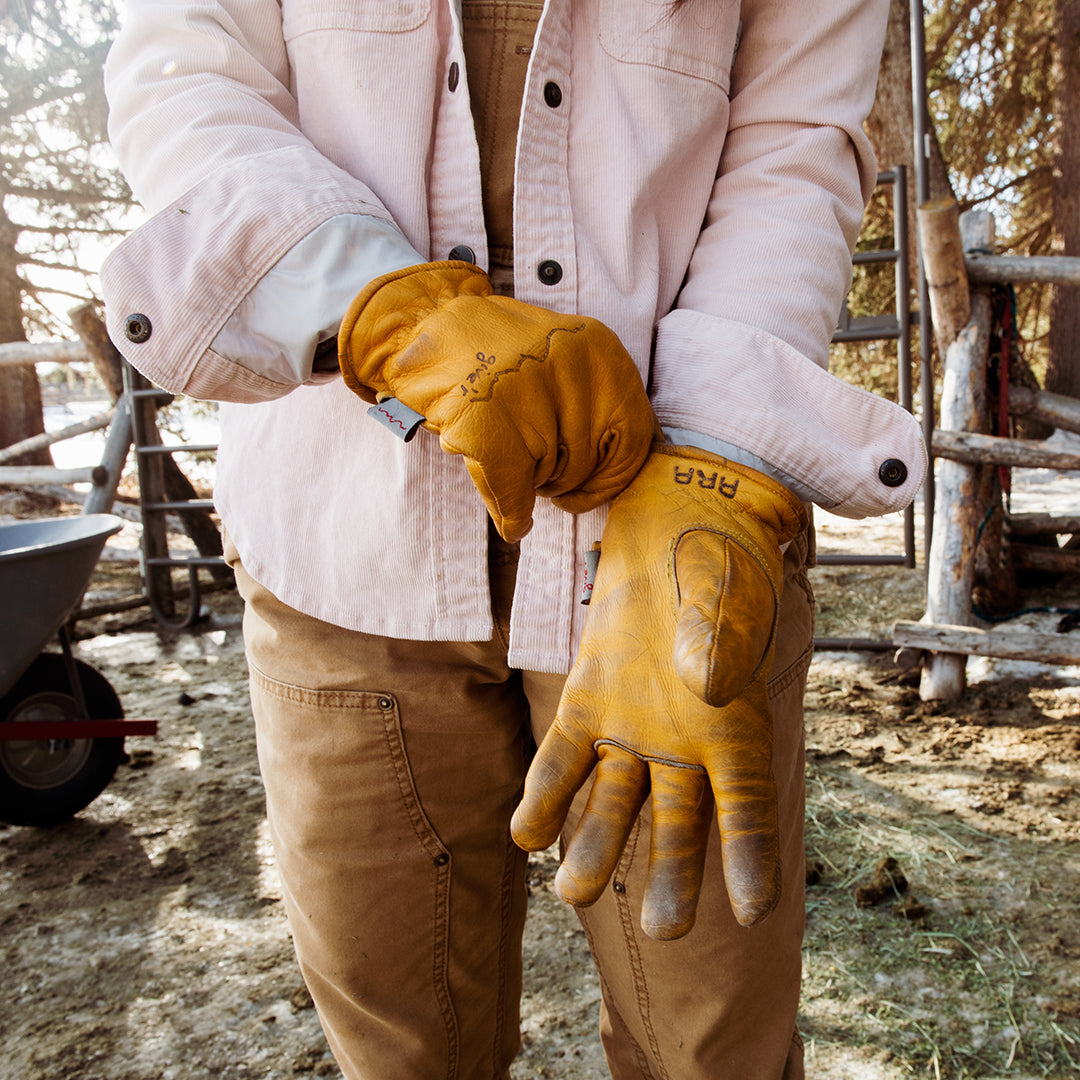A person is standing outdoors, seemingly in a fenced-in area with a natural, slightly cluttered ground covered in dirt, hay, and alfalfa. The individual is actively putting on a pair of well-worn leather gloves. The right glove is facing downwards, with brown-colored fingers and the initials "RRR" inscribed near the wrist. Their left hand, with fingers curled together, pulls up the right glove, revealing a gray tag with an amber squiggly line.

The person is dressed in a light pink long-sleeve jacket adorned with black buttons, and paired with khaki-colored, possibly work-style pants featuring pockets. The attire suggests they might be engaged in some form of outdoor labor.

In the background, to the left side of the image, is a portion of a wheelbarrow with a black tire. On the right side, a wooden fence made from logs, attached to a metal gate, is visible. The scene is further enriched by a blurred backdrop of trees, indicating a forested setting with the sunlight casting shadows, adding depth and texture to the environment.